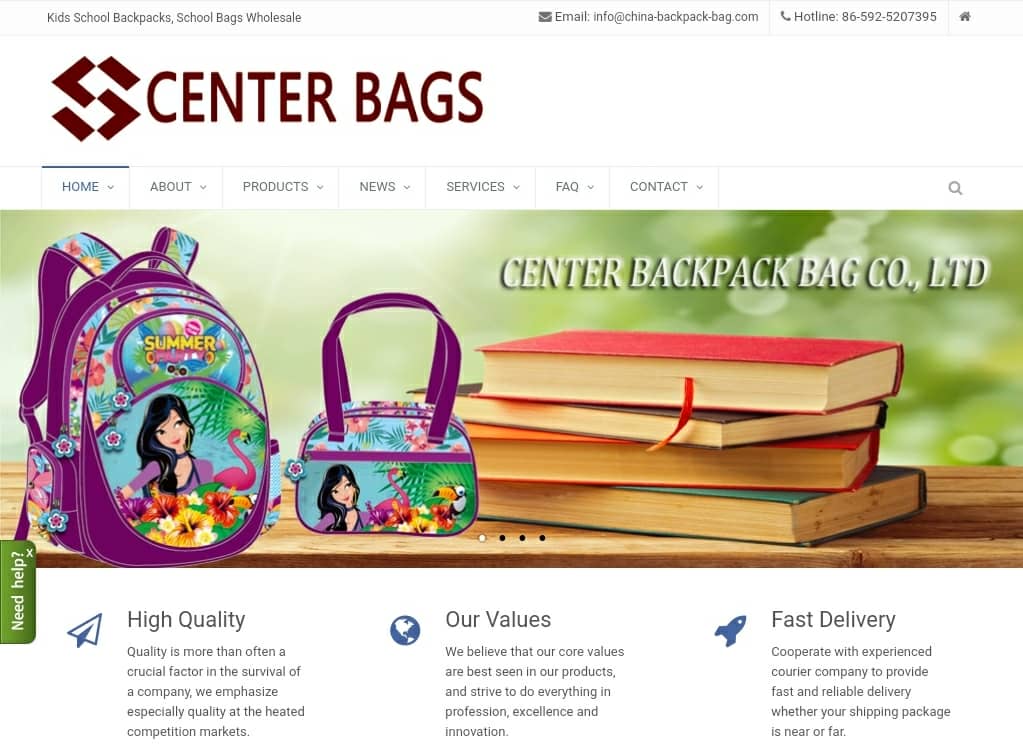The image captures a detailed view of a website page for Center Bags. At the top left, in dark maroon text, the business name "CENTER BAGS" is prominently displayed alongside a logo resembling an angular, broken letter S. To the right, contact information is neatly organized with an envelope symbol followed by the email "info@china-backpack-bag.com" and a phone icon next to the hotline number "+86-592-5207395." A home icon is also situated here. The navigation menu sits just below, offering tabs for Home, About, Products, News, Services, FAQ, and Contact, each adorned with a downward-pointing triangle for dropdown options and a magnifying glass symbol for search functionality.

In the center of the webpage is an illustrative image featuring a colorful, cartoon-style backpack and handbag adorned with images of a girl, a flamingo, and flowers, accompanied by the text "Summer Hut." Beside these items, a stack of four books in red, brown, red, and green can be seen, with the top book showcasing a red bookmark. Floating above this visual arrangement, in white capital letters, is the inscription "CENTER BACKPACK BAG CO., LTD."

Lower on the page, three icons accompanied by detailed explanatory text emphasize the company's commitment to high quality, core values, and fast delivery. An envelope icon introduces the high quality section, highlighting the importance of quality in competitive markets. A globe icon describes the company's values—professionalism, excellence, and innovation. Finally, a rocket icon discusses the company's partnership with experienced couriers to ensure swift and reliable delivery. Just beside these items, a green rectangle with sideways text queries, "Need help?" followed by a small "X" symbol.